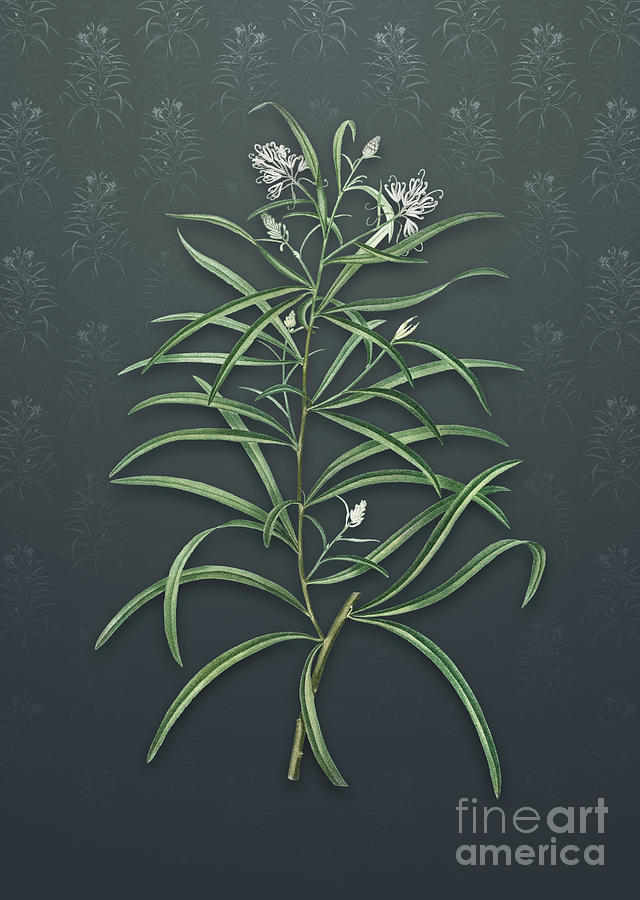This is an image of a vividly detailed, leafy plant with long, thin, wispy green leaves resembling spider legs, centered against a dark grey backdrop. The plant features delicate, lace-like white flowers at the top, with a couple of additional flowers emerging from the middle. The leaves exhibit fine white or yellow lines, adding to the texture. The background transitions from a solid dark grey in the bottom half to a faint repeating plant pattern at the top, creating a visually dynamic effect. The replicated plants are more faded, contributing to the layered depth of the artwork. The overall composition is dark and moody, with no frame or border, and in the bottom right-hand corner, the text reads "Fine Art America."